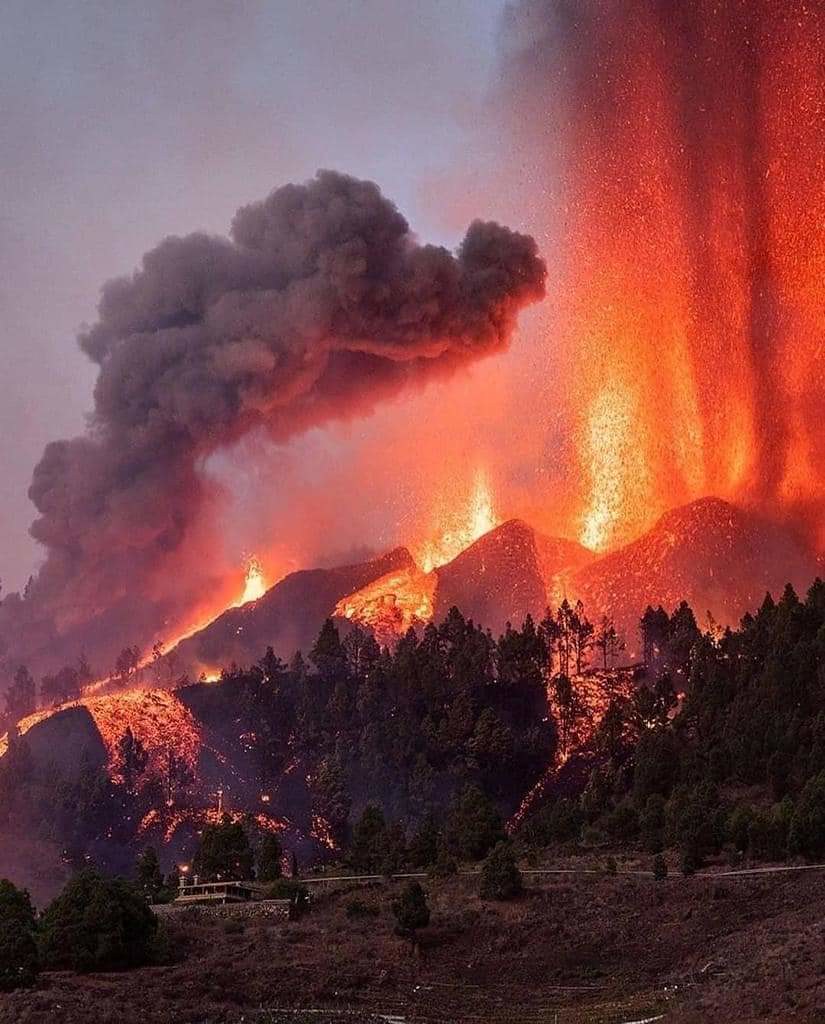The photograph depicts a dramatic landscape dominated by a volcanic eruption. In the foreground, a small house and road are barely visible amidst the dark, forested area at the base of a towering mountain. The lush greenery gradually gives way to fiery chaos, with vibrant red, yellow, and orange lava flows cascading down the slopes, setting the forest ablaze. Several intense fires are scattered across the mountainside, sending columns of bright, glowing lava upward. The eruption is accentuated by a massive plume of black smoke on the left side, transitioning to lighter shades of gray and red as it ascends. The right side of the frame is consumed by the raging volcano, which stretches from the middle to the top of the photo, with its dark, molten core vividly clashing against the inferno of orange and yellow lava. The scene is both mesmerizing and devastating, capturing the raw power of nature's fury.